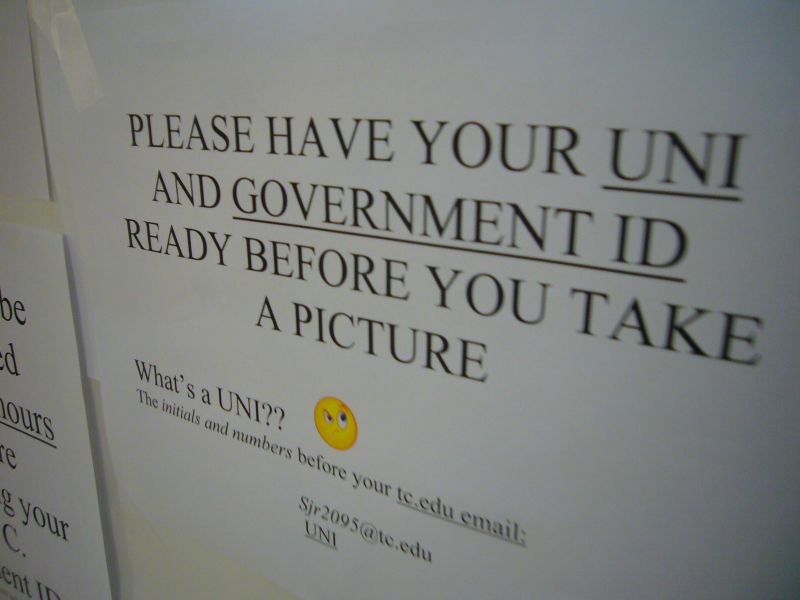The image depicts a white paper sign affixed to a billboard or wall, secured with sellotape at the top left corner. The sign is filled with a series of directions and clarifying notes, all in black text on a white background. The main instruction, which is underlined for emphasis, reads: "Please have your UNI and government ID ready before you take a picture." Below this instruction, another underlined text states, "What's a UNI?" next to a puzzled yellow emoji. Following the emoji, the text explains: "The initials and numbers before your tc.edu email." Finally, the sign is signed off with "sjr2095@tc.edu" and the acronym "UNI" underlined again. There's an additional smaller, similar white paper sign with black text positioned at the bottom left of the image. This setup suggests the sign is located in an educational setting, likely a college, indicating that it pertains to the process of obtaining a student ID.